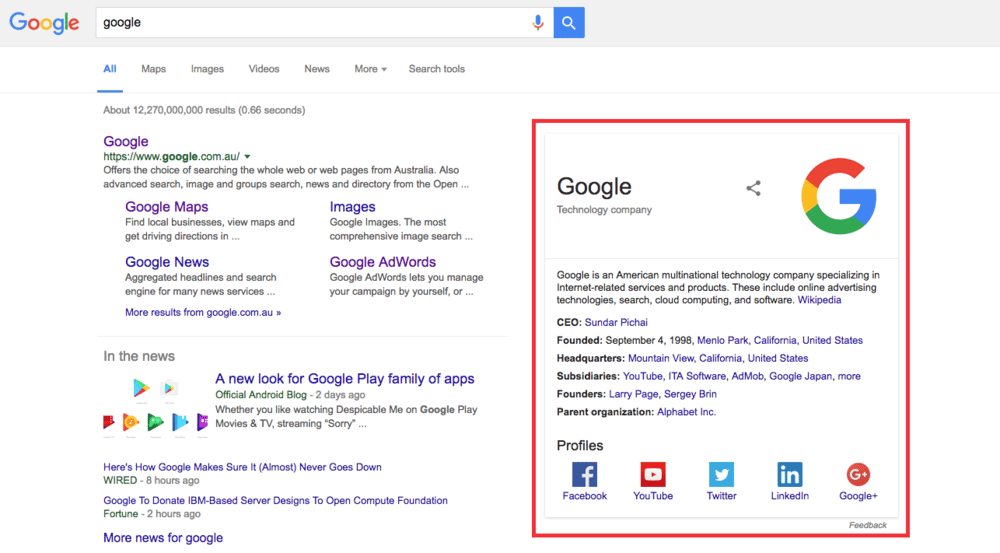The image depicts a clean, white background with Google’s search interface prominently displayed. At the top, the familiar Google logo is situated above a search bar which contains the word "Google". The search bar features a microphone icon on the right side and a blue square with a white magnifying glass symbol at the far right. Below the search bar, the navigation links “All,” “Maps,” “Images,” “Videos,” “News,” “More,” and “Search tools” are underlined in blue.

Further down, there’s a section showcasing search results for "Google". A green web address reads "google.com" followed by several related categories like “Google Maps,” “Google Images,” “Google News,” and “Google AdWords.” Additionally, there are news snippets such as "A new look for Google Play family of apps - Official Android Blog - 2 days ago” and "Here's how Google makes sure it (almost) never goes down - Google to donate IBM base server designs to Open Compute Foundation." Also highlighted in green is “More news for Google.”

In the bottom left corner of the image, a red outline encloses detailed information about Google. This includes "Google - Technology Company" mentioned twice. It provides information about Google’s CEO Sundar Pichai, the date founded which is September 4, 1988, and lists the headquarters’ information along with details about subsidiaries and founders, Larry Page and Sergey Brin.